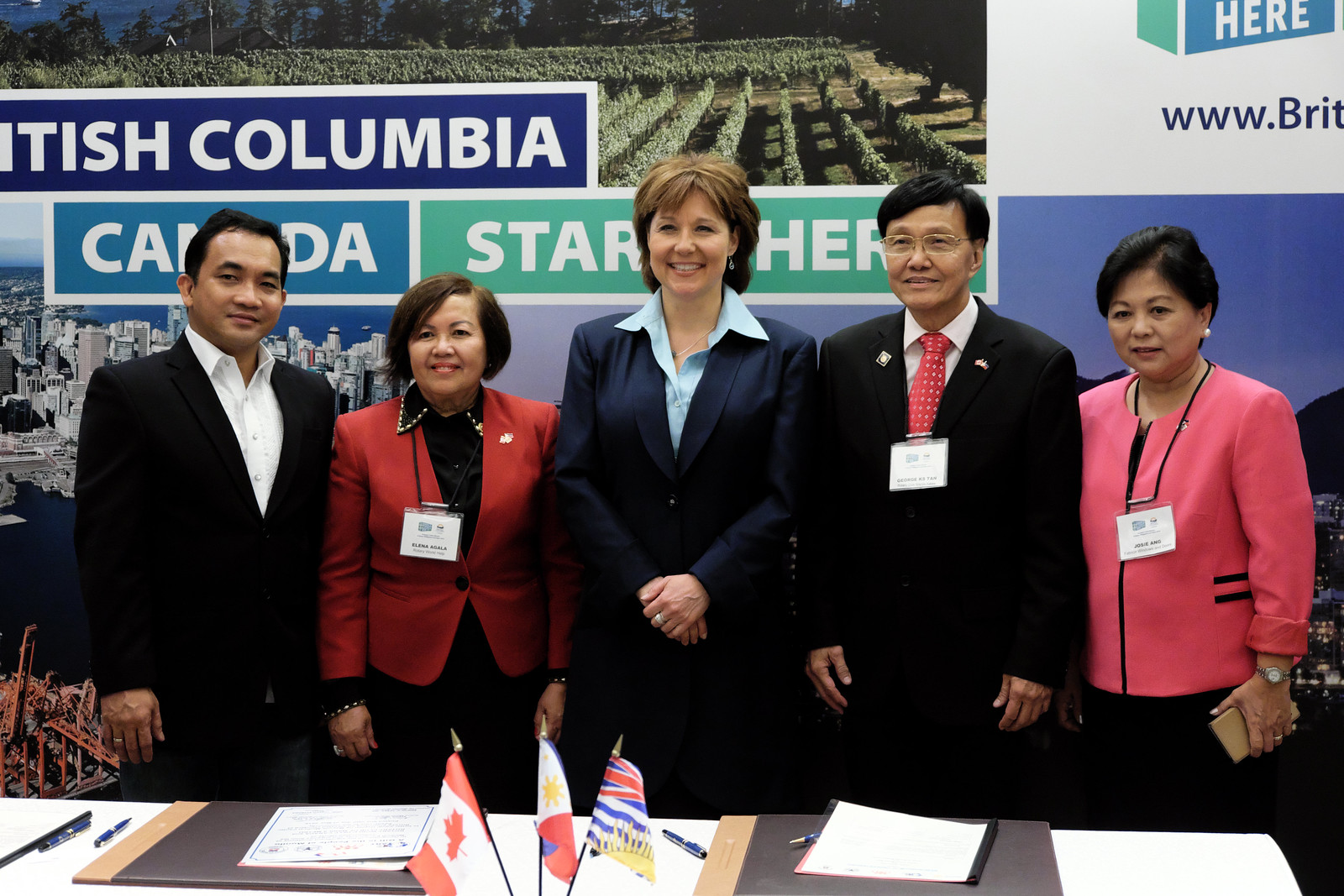This photograph captures a vivid scene of five individuals standing shoulder to shoulder, smiling, and posing for the camera. They stand behind a low table adorned with various papers, ink pens, and three small flags representing Canada, Great Britain, and the Philippines. The background features a large poster with images depicting scenic green fields, large buildings beside a blue water body, construction equipment, and a city skyline illuminated at night. The headline on the poster reads "British Columbia, Canada. Start Here," accompanied by a logo and partial web address.

From left to right, the individuals are:
- A man with short dark hair, wearing a black suit jacket and white shirt.
- A shorter woman in a red jacket, black top, and black pants with an ID card around her neck.
- A tall woman with short brown hair, dressed in a navy blue blazer, light blue shirt, and black pants, wearing a ring on her finger.
- A man of similar height with short black hair, clean-shaven, outfitted in a black suit, white shirt, red tie, glasses, and an ID card around his neck.
- A shorter woman in a pink jacket, holding a mobile phone, wearing a wristwatch, black pants, ear studs, and an ID card around her neck.

The arrangement of the individuals and the detailed setting behind them suggests they are part of a formal event or conference, possibly promoting opportunities in British Columbia, Canada.